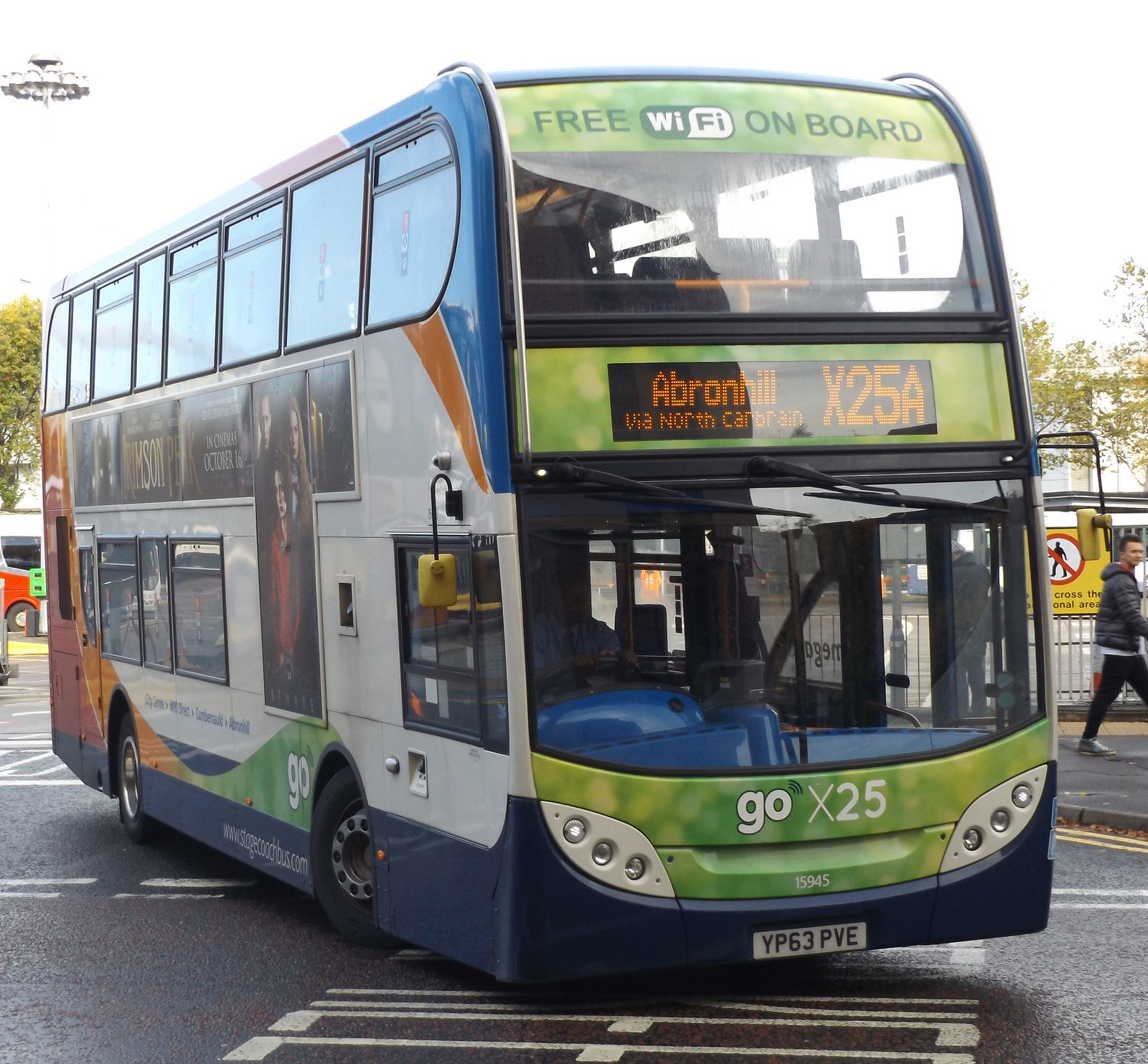In the image, a double-decker bus takes center focus as it sits on a gray street markedly lined with white and yellow road markings. The bus, prominently numbered 15945, features "GO" and "X25A" on the front, along with a license plate reading YP63PVE. The front also boasts six lights and an advertisement for "Crimson Peak" or a similar entity.

On the right side of the frame, a man dressed in a jacket and black pants is seen walking away from the bus. The bus displays an intricate array of details: its two levels are visible through large windows, showing rows of blue seats and various other seats on both decks. A large, clear driver's window reveals the steering wheel and additional interior seating. The top deck is adorned with a "Free Wi-Fi on board" banner, indicating passenger amenities. Further along the side, more windows allow glimpses into both levels, with advertisements and images of people situated beneath the upper deck windows. The bus also features a partly legible website along its lower edge.

On closer inspection, no bus driver or passengers are evident, suggesting the bus might be stationary, either parked or awaiting passengers.